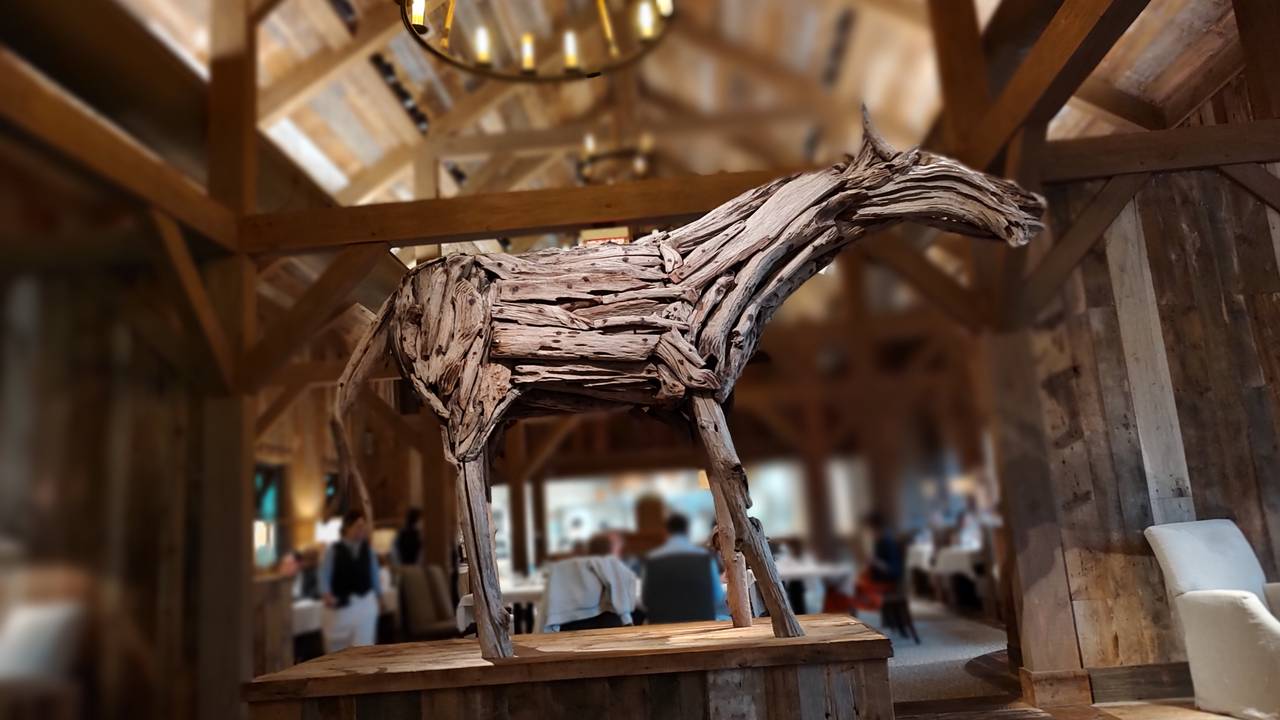The image features a detailed close-up of a wooden horse statue, skillfully assembled from twigs and wood shavings, giving it an intricate, textured appearance. The horse stands on a brown wooden platform and faces to the right, characterized by an elongated neck and head. The background reveals a rustic, restaurant setting with abundant brown wood, reminiscent of a barn structure. There are exposed wooden beams, board walls, and a wagon wheel chandelier contributing to the decor. Blurred tables with white tablecloths and patrons, some of whom are dressed in black vests and white pants, are visible in the background, enhancing the ambiance. Further details include a light blue business suit worn by a server and an upholstered white chair to the bottom right, adding subtle elegance to the scene.